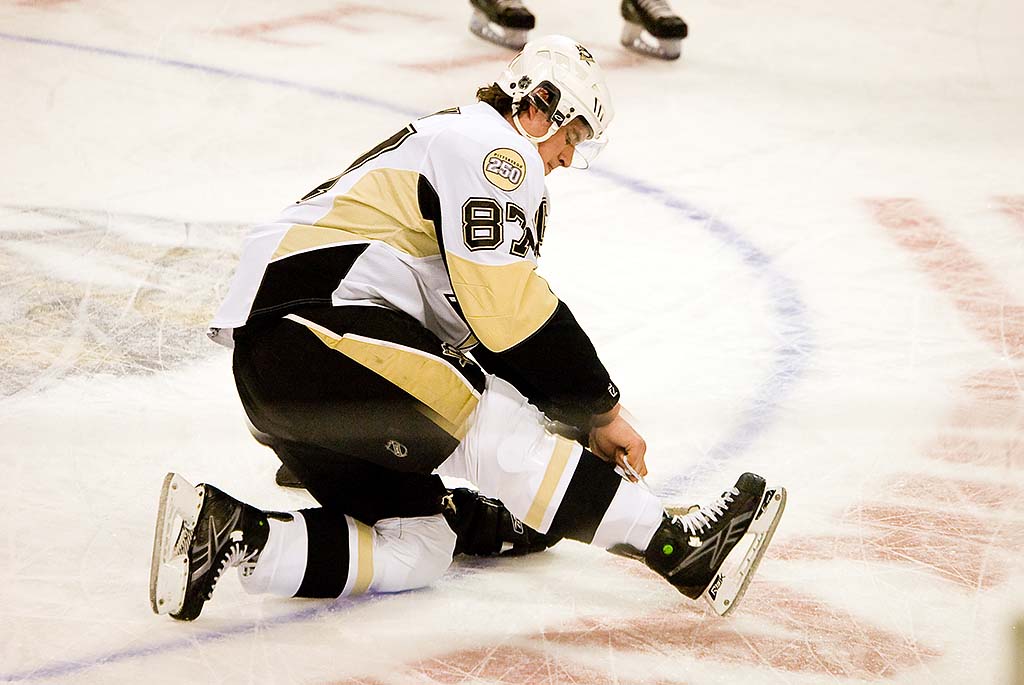In this detailed photograph from a hockey game, a player wearing a black, gold, and white uniform with the number 87 and a "250" patch on his right shoulder is kneeling on the scraped-up ice. He's positioned with his left knee down and his right leg extended, facing towards the right side of the image. The player, a white male with dark hair, is adjusting his black Reebok skates, identifiable by the gray Reebok symbol and white bottoms. His uniform features intricate detailing with white, yellowish-tan, and black on the top, and black pants with gold, white, and tan stripes. The ice, marked with red writing and blue circular areas, suggests the game has been ongoing for some time. In the background, partially visible, are the skates of another player moving towards him. The photograph captures a moment of possible discomfort or equipment adjustment during an intense game.